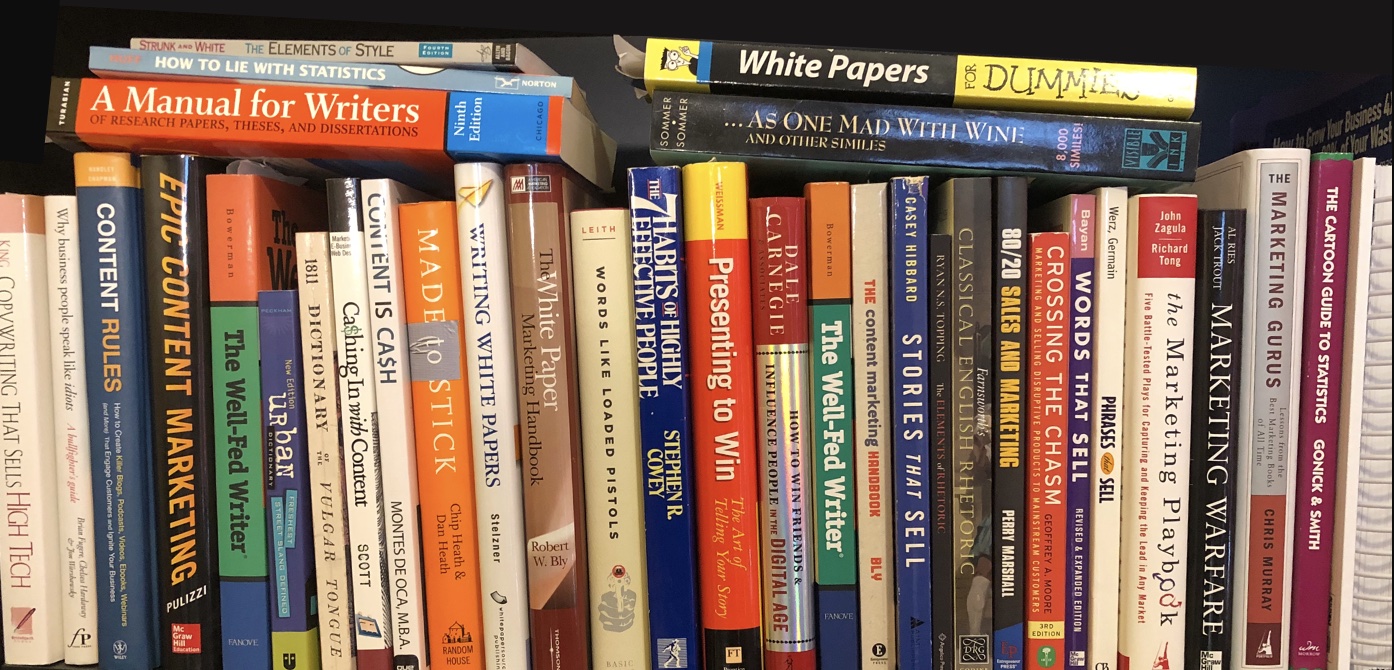This vibrant, color-filled photograph captures a well-organized bookshelf presumably belonging to a writer or a scholar. The shelf is densely packed with a variety of titles primarily focusing on writing, marketing, and presentation skills. The books are mostly standing vertically with their spines facing outward, displaying titles like "A Manual for Writers" and "Presenting to Win." These are interspersed with horizontally stacked books such as "White Papers for Dummies" and "Content Rules". Notably, there are two copies of "The Well-Fed Writer" featured prominently. Other titles include "Words that Sell," "The Marketing Playbook," and Stephen Covey's "The Seven Habits of Highly Effective People." The books vary widely in color and size, with vibrant hues such as the orange cover of "A Manual for Writers" and the yellow and black "White Papers for Dummies." The image effectively illustrates a curated collection of resources essential for honing writing and presentation skills.